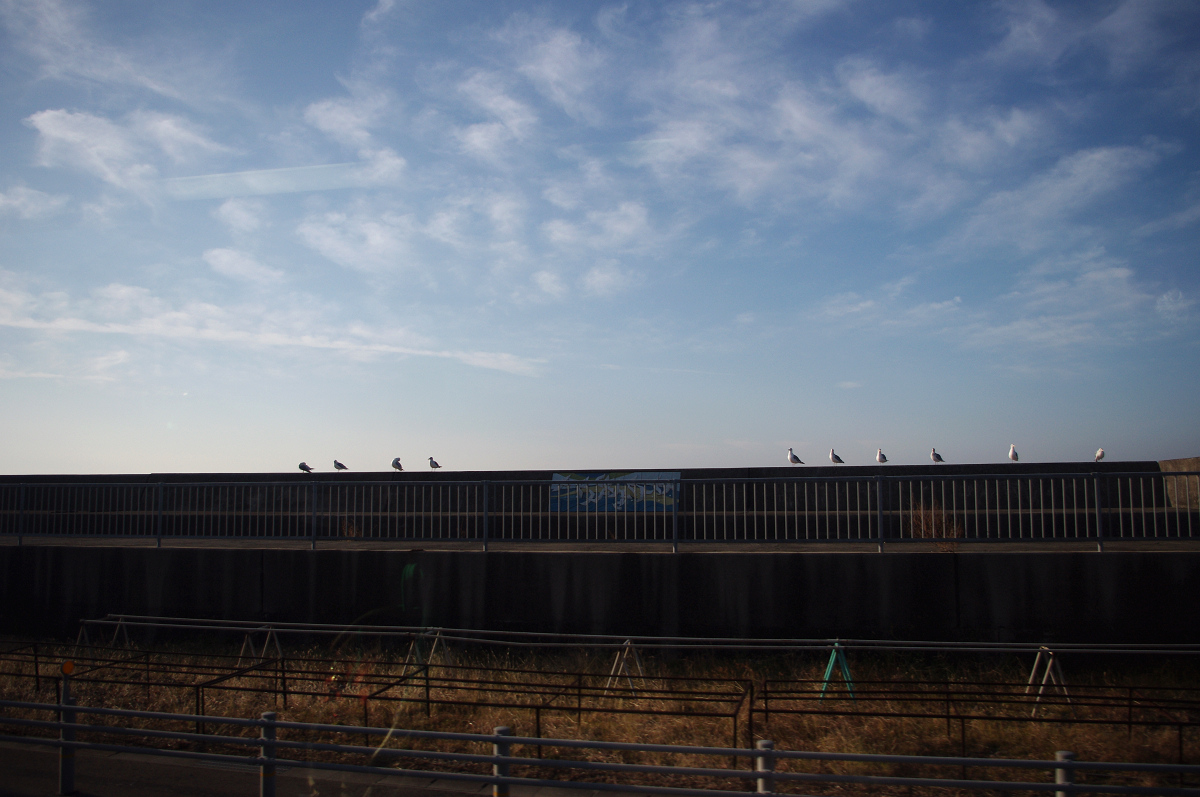The photograph captures a distant view of a rustic structure, potentially a building or a water system, occupying the lower half of the image. The structure features a vinyl label or poster prominently displayed in its center. Its top is crowded with birds, mostly seagulls and pigeons, perched on both the left and right sides. The foreground appears dark due to the shadows, showcasing layers of pipe fencing atop triangular supports, and a partially visible damaged grassy area, likely scorched by the sun. The backdrop is a bright blue sky with high, thin, light clouds, creating an overhazed look that silhouettes the birds against this serene setting. Beneath the structure runs a rusty wrought iron railing and additional fencing, providing a stark contrast with the vibrant sky above.